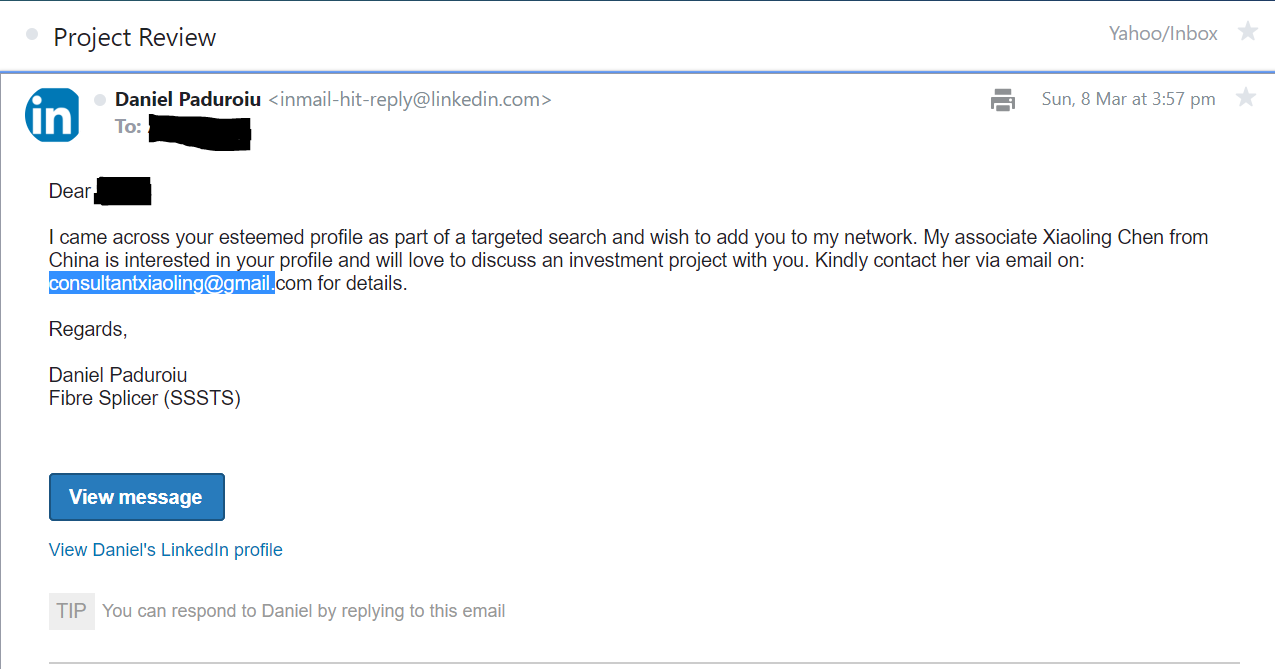Here’s a detailed and cleaned-up caption:

---

This image captures a screenshot of an email received in a Yahoo inbox. The subject line reads "Project Review," and the email is a LinkedIn notification from Daniel Paduroiu (email: hit-reply@linkedin.com). The message, sent on Sunday, March 8th at 3:57 p.m., addresses the recipient with "Dear [Name]," which is obscured. Daniel states that he came across the recipient's esteemed profile during a targeted search and wishes to connect on LinkedIn. He mentions his associate, Xiaoling Chen from China, who is interested in discussing an investment project. The recipient is advised to contact Xiaoling via her email, consultantxiaoling@gmail.com, for more details. The email concludes with Daniel's signature, listing his role as a Fiber Splicer at S-S-S-T-S. 

The recipient has previously messaged Daniel on LinkedIn.

---